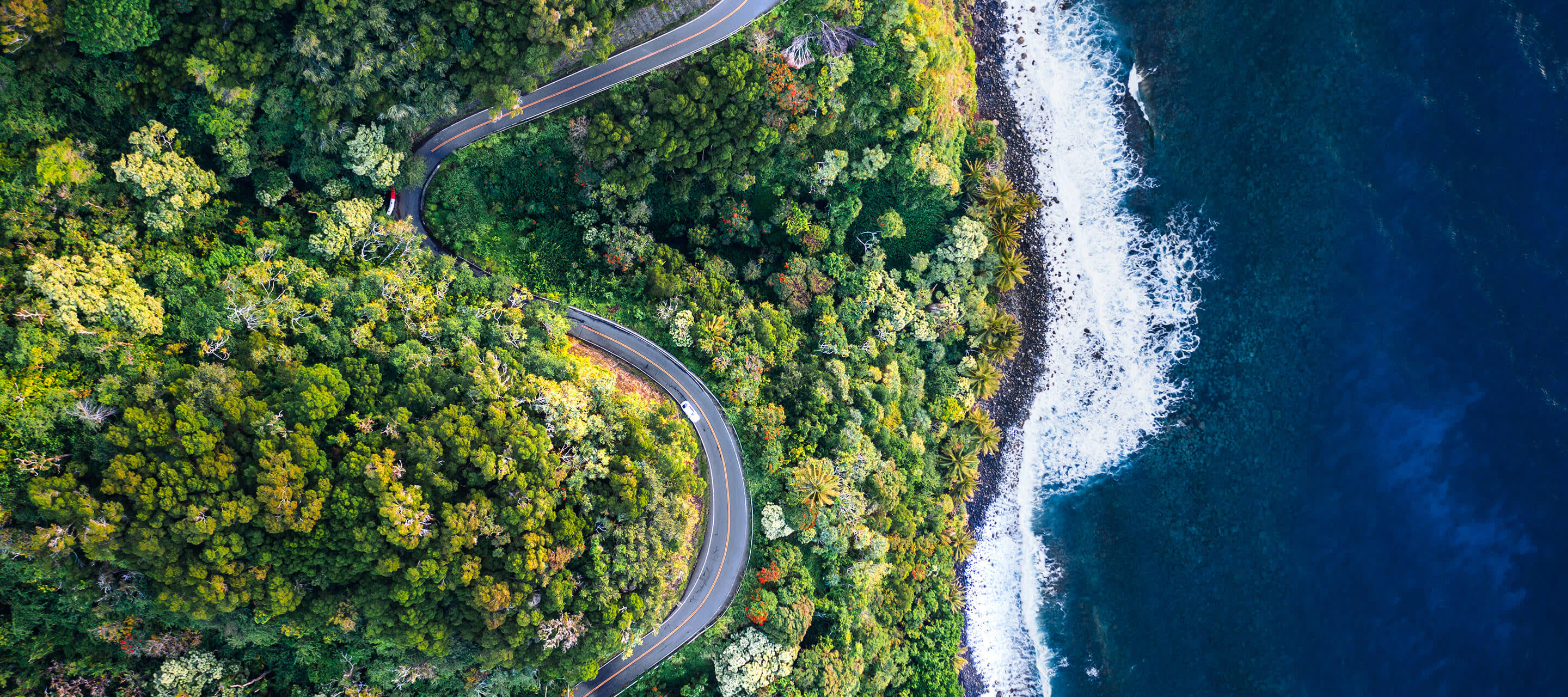The image is a full-color aerial photograph with a rectangular shape, oriented horizontally. It captures a winding, two-lane highway with a yellow stripe down the middle, snaking its way through a densely wooded area adorned with various shades of green foliage. This vibrant forest occupies most of the left side of the image. Two vehicles are visible on the road—one is white, and the other is red and white. To the right of the highway, a striking blue body of water meets a rocky shoreline, marked by white caps where the waves crash against the shore. The shoreline runs almost the entire vertical length of the image, providing a dynamic contrast between the lush greenery and the expansive, vibrant ocean. The highway itself follows an S-shaped path through this picturesque landscape, seamlessly blending the terrestrial and aquatic elements of the scene.